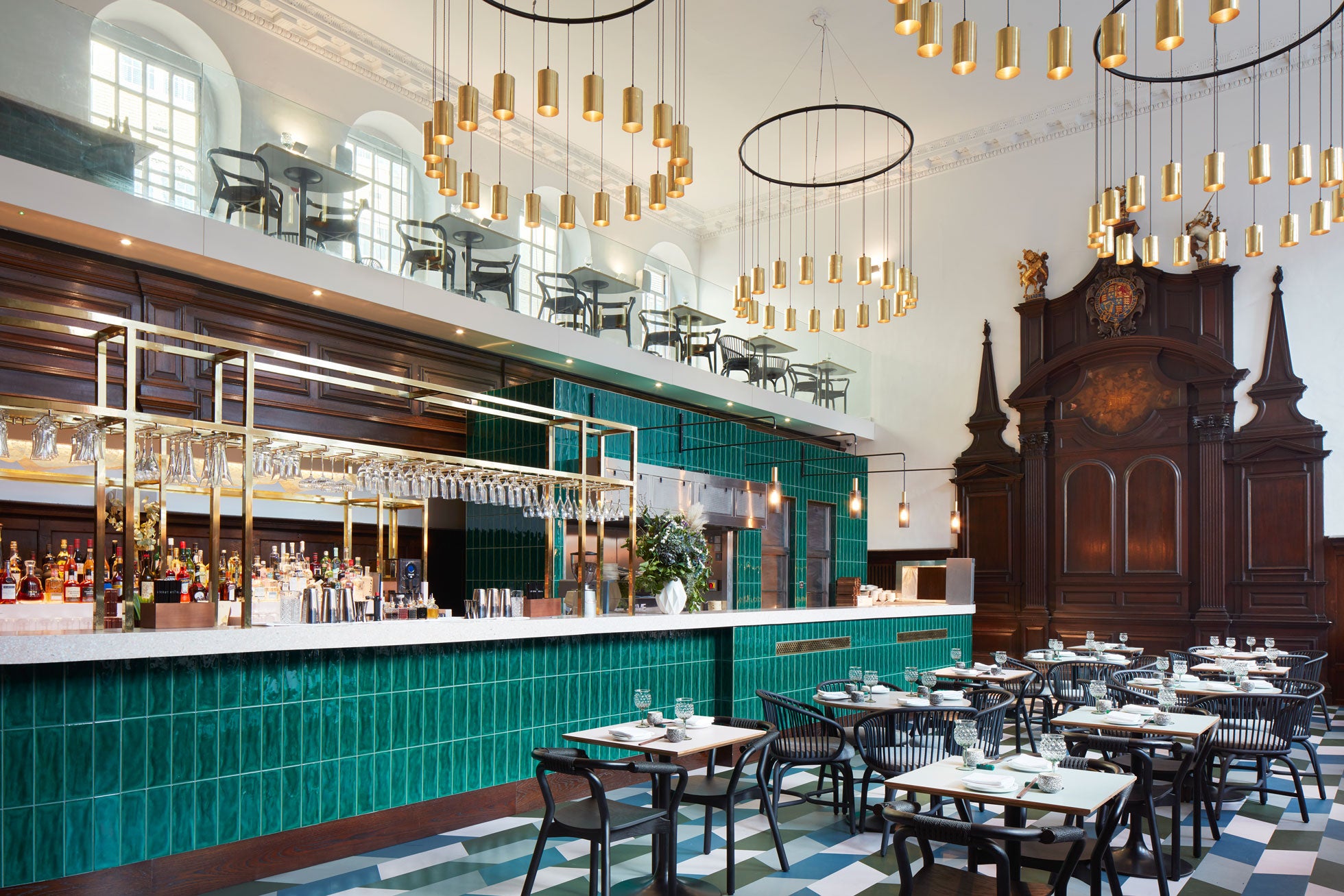This image showcases an elegant, upscale cocktail lounge that exudes sophistication and charm. The long bar gleams with turquoise-green tiles set in white mortar, topped with a pristine white countertop. Brass rails adorn the top, from which a variety of glasses – martini, rock, wine, champagne – hang elegantly. On the bar, below the glassware, lie the standard accouterments of a well-stocked bar - shakers, bottles, and other tools of the trade. The foreground is dotted with a mix of circular and rectangular tables, each set with black chairs and white tops, beautifully arranged with dinette sets including plates and wine glasses, laid out on a stunning blue, white, and black mosaic tiled floor.

The lounge's back wall is dominated by a grand, ornate wooden structure that reaches impressively high, reminiscent of a church steeple or an altarpiece, set against a pristine white wall. Above the main bar area is a second-floor seating area with a balcony lined with a glass railing, offering an elevated perch for patrons. This upper area mirrors the setup below with matching tables and chairs. Massive windows behind the balcony flood the space with natural light, enhancing the room's spacious ambiance.

Suspended from the towering white ceiling are four spectacular chandeliers. Each chandelier features a circular arrangement from which about twenty golden light fixtures extend, casting a warm and inviting glow throughout the space. The overall atmosphere of this sophisticated lounge is accentuated by its open, airy feel and careful attention to detail in décor and furnishings.